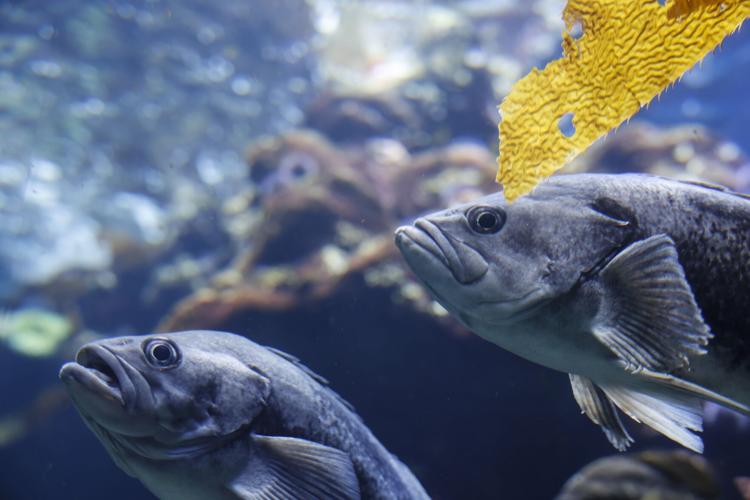This underwater photograph features a close-up view of two bluish-gray fish, with only the front halves of their bodies visible. Both fish are positioned with one towards the left and the other towards the right, seemingly swimming side by side. The fish on the left has its mouth slightly open, while the fish on the right has its mouth closed. They both have circular eyes.

In the upper right corner of the image, there's a yellow object that might be a piece of seaweed or a leaf, adorned with some brown lines. The background of the photograph is slightly blurred, predominantly blue in color, and includes some indistinct elements such as a brown rock-like structure and bubbles. There also appears to be a suggestion of other aquatic life, with out-of-focus shapes that might include more fish or possibly even an octopus.